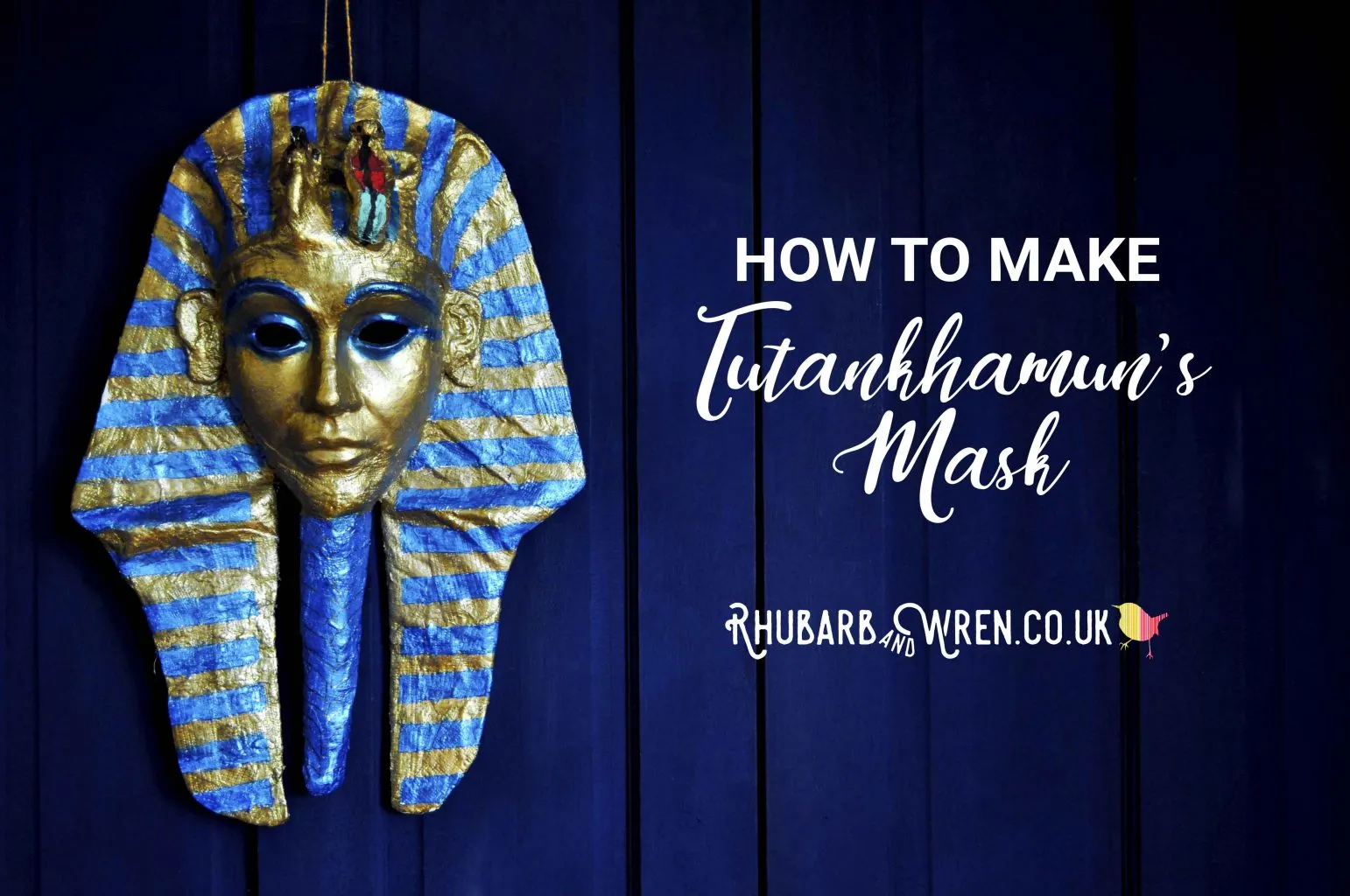The image features a poster against a deep royal blue, pleated curtain. On the right side, in white text, it reads "How to Make Tutankhamun's Mask." Below this text is the URL "rhubarbandwren.co.uk" accompanied by a pink and peach bird logo. To the left, there's an elaborate Egyptian mask, possibly representing King Tutankhamun. The mask is predominantly gold with a striking blue and gold striped headdress, known as a nemes, that alternates blue and gold stripes encompassing the face. The golden face has blue detailing around the eyes and eyebrows, with a notable blue stripe extending from the chin. The mask is richly adorned, capturing the opulence and regal essence of ancient Egyptian royalty, set against the elegant backdrop of the blue curtain.